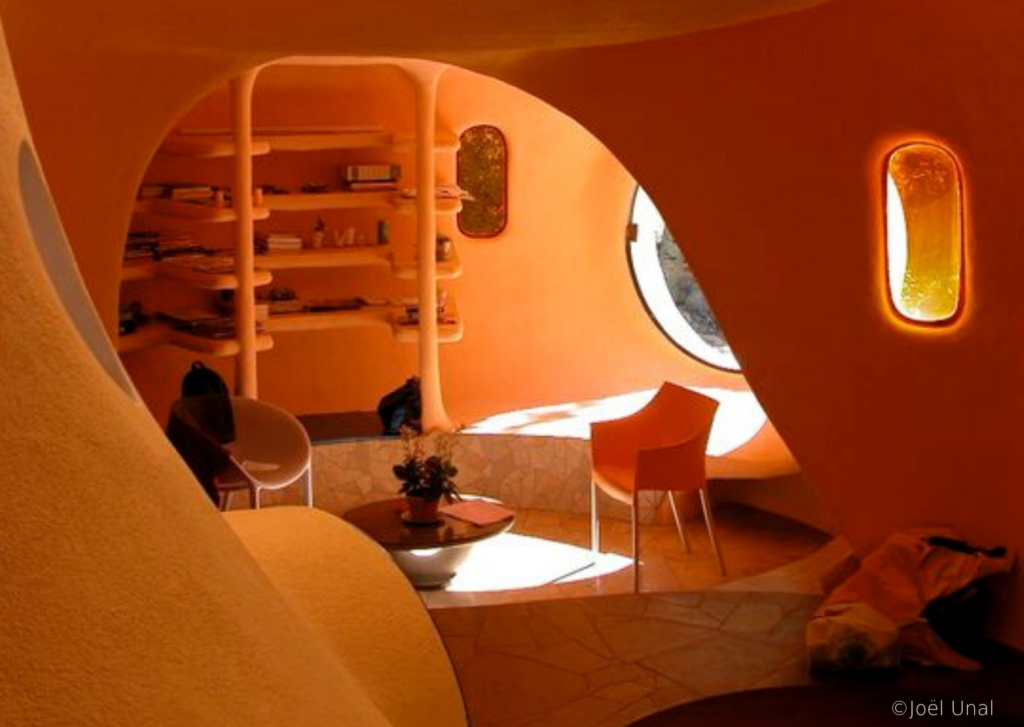The photograph showcases the interior of a distinctive, modern dwelling with organic, earthship-style architecture characterized by rounded, stucco-like walls and ceilings. The predominant color throughout the room is a warm, orange hue, which covers the textured walls and contributes to the cozy, inviting atmosphere. Central to the room is a small, circular, recessed chatting nook with a round table, adorned with a flower arrangement and a few potted plants, accompanied by a couple of chairs, including one distinctly orange chair. The stone-tiled floor, consisting of various shapes, adds to the earthy aesthetic. A circular window on the right side allows abundant daylight to stream in, illuminating the space and offering a view of an outdoor rock formation. Towards the back, there's a recessed area near the round window, which could serve as a ledge or possibly even a bed. In the background, a modern-looking bookshelf, seemingly crafted from the same clay-like material as the walls, holds an assortment of books and knick-knacks. The photograph, which includes a watermark in the bottom right-hand corner reading "Joel Unal" with a copyright symbol, is wider than it is tall, measuring approximately six inches wide and four inches high.